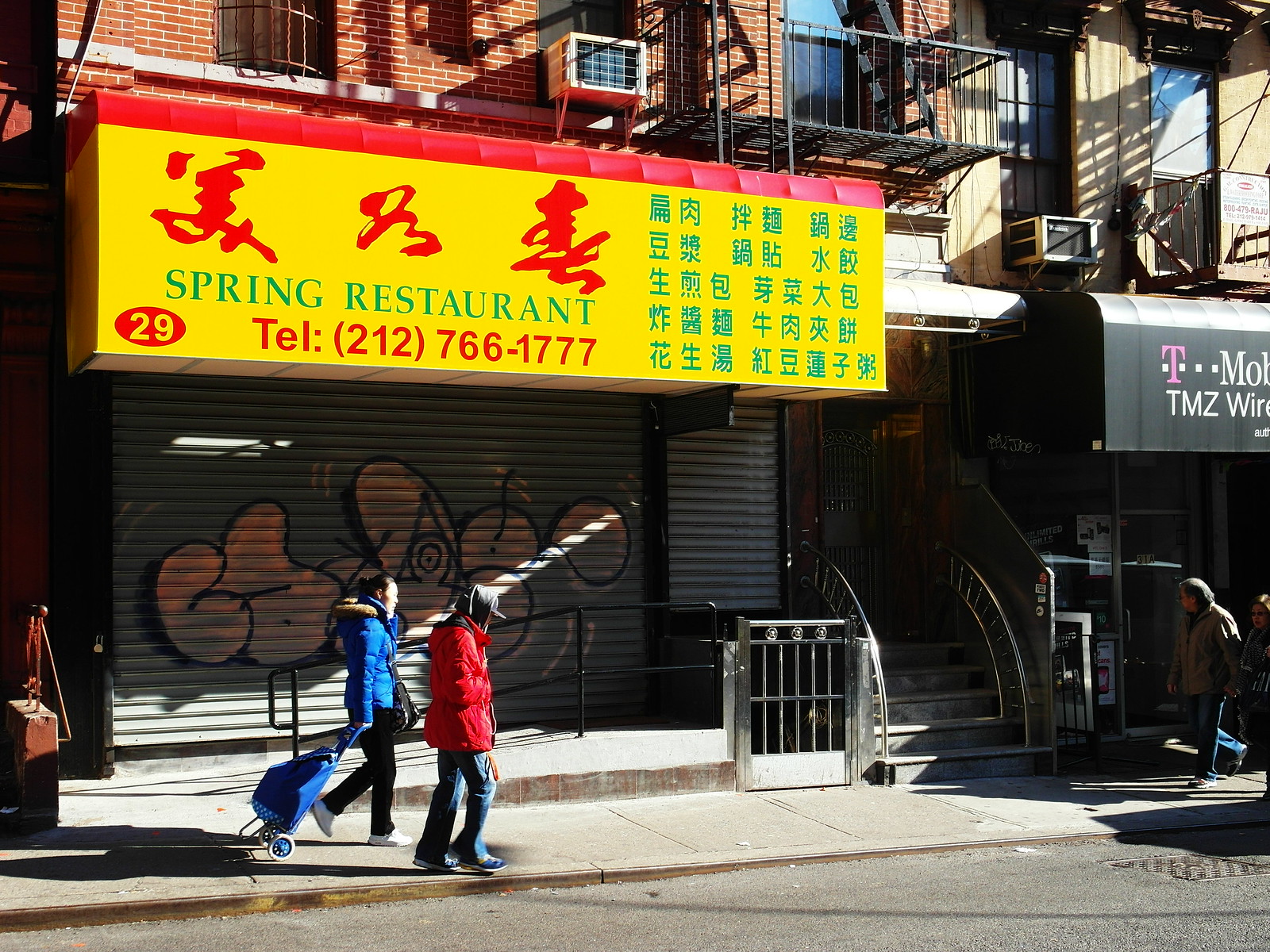This photograph captures an urban street scene during the daytime, in front of a closed storefront identified as "Spring Restaurant." Prominent on the storefront is a large yellow sign with red and green Asian characters, and below these, the words "Spring Restaurant" are displayed in green, along with the telephone number 212-766-1777. The sign also features a red oval with the number 29 in it. The storefront is secured with a grey steel panel, which is covered in graffiti.

In the foreground, two people walk on the sidewalk. The woman on the left is dressed in a blue parka, black pants, and white sneakers, and she's dragging a blue suitcase on wheels. Beside her, a man wears a red parka, a hoodie, a baseball cap, blue jeans adorned with a red keychain, and blue sneakers. Heading in their direction, a third person—a man in a brown jacket and blue pants—walks toward them.

Above the storefront, the building shows signs of residential apartments with visible windows and an air conditioning unit. To the right of this scene, there is a black awning with the T-Mobile logo, part of a neighboring store. The sun shines brightly, casting shadows and highlighting the busyness and layered details of this typical cityscape.